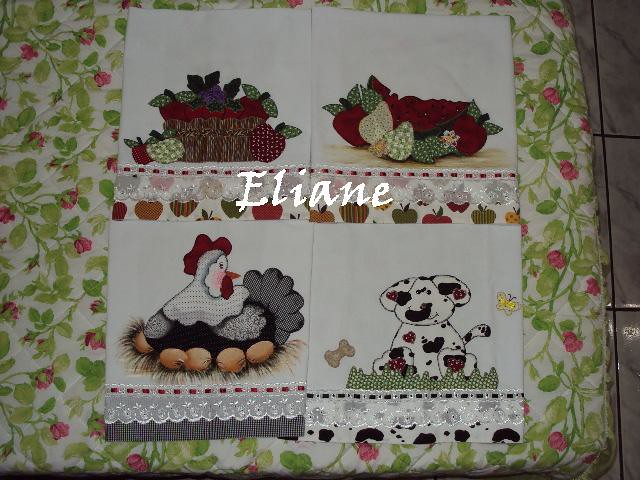This image features four distinct and intricately designed tablecloths displayed over a quilted white tablecloth adorned with sprawling pink roses and predominantly green leaves. The scene is set against a white tile floor. Each tablecloth is unique in design:

- The top left tablecloth showcases a fruit basket filled with strawberries and apples, enhanced with a lace border.
- The top right tablecloth displays a variety of quilted-style fruits, including watermelon, also accented with lace.
- The bottom left tablecloth features a chicken with a black body, gray wings, a white head and neck, and red combs, sitting near five eggs on a black and white checkered pattern with a lace border.
- The bottom right tablecloth depicts a white dog with black spots, decorated with red hearts, a butterfly, a bone, and green swirls representing grass, all framed by a lace pattern.

In the background of the image, embroidered on the quilted tablecloth, is the name "Elaine" in white, tying together the richly detailed presentation.